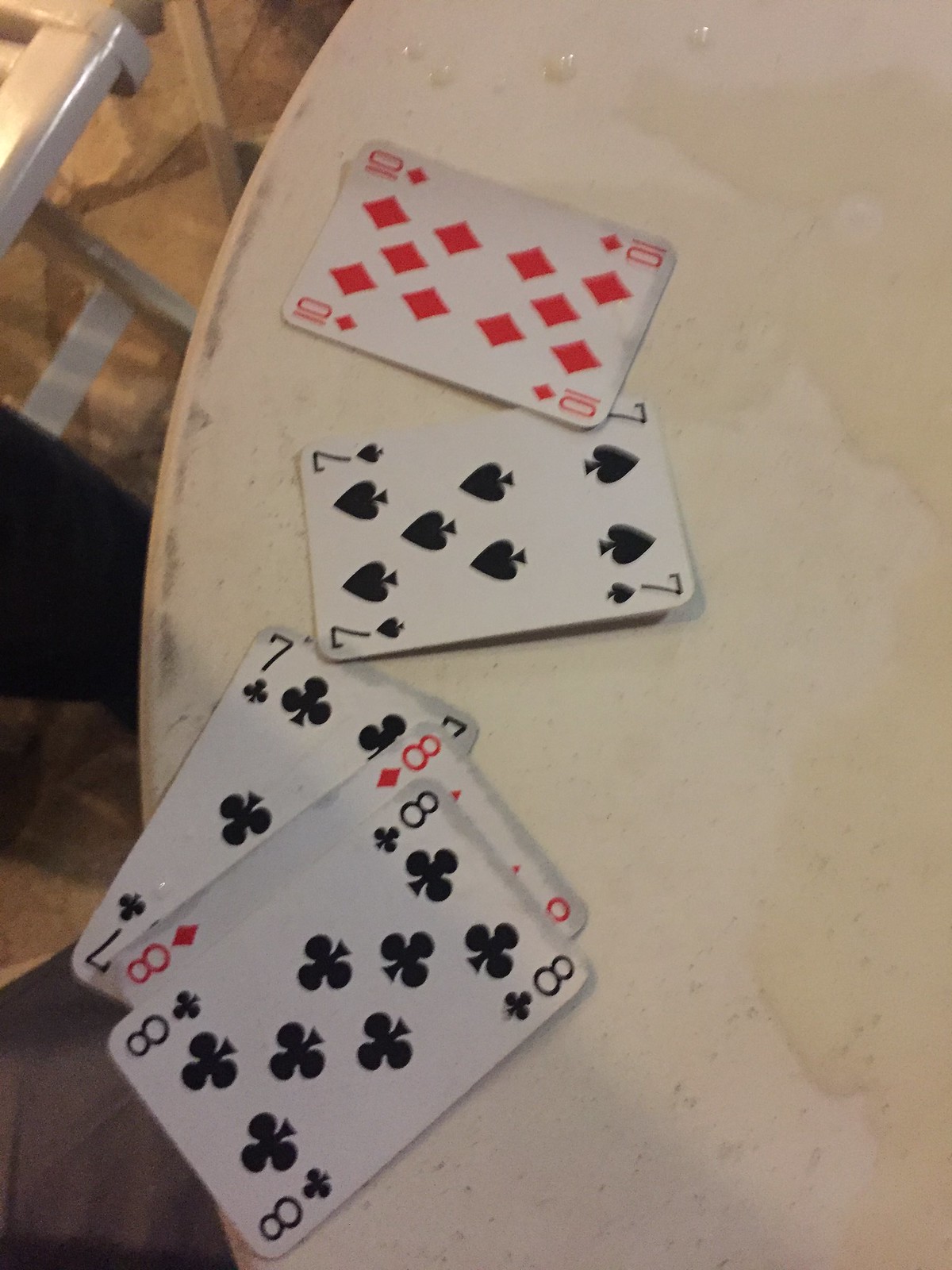In this vibrant color photograph, a dirty, white, circular table is prominently featured, riddled with various stains and active spills, hinting at recent use. A light yellow liquid appears to be the latest culprit, seeping across the tabletop and affecting a set of playing cards. The cards are arranged haphazardly: at the top lies a 10 of Diamonds and a 7 of Spades, while below them, a 7 of Clubs, 8 of Diamonds, and 8 of Clubs cluster together, noticeably soaked by the spillage. To the upper left, a white foldable chair partially enters the frame, suggesting a casual or impromptu setting. The ground beneath the scene is a warm brown, contrasting with the chaotic tableau above.